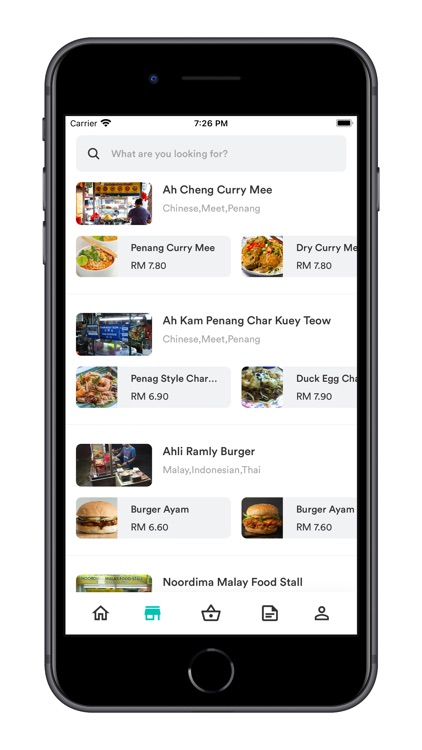The image depicts a smartphone displaying a food ordering webpage. At the top of the screen, there is a search button allowing users to easily find specific dishes. Below the search button, the webpage showcases various culinary selections categorized by cuisine types including Chinese, Malay, Indonesian, and Thai. The page displays appetizing images of each dish, with options like Penang curry, dry curry, Penang-style chicken, and duck egg prominently featured. Users can scroll through these mouth-watering selections and choose their desired meal effortlessly.